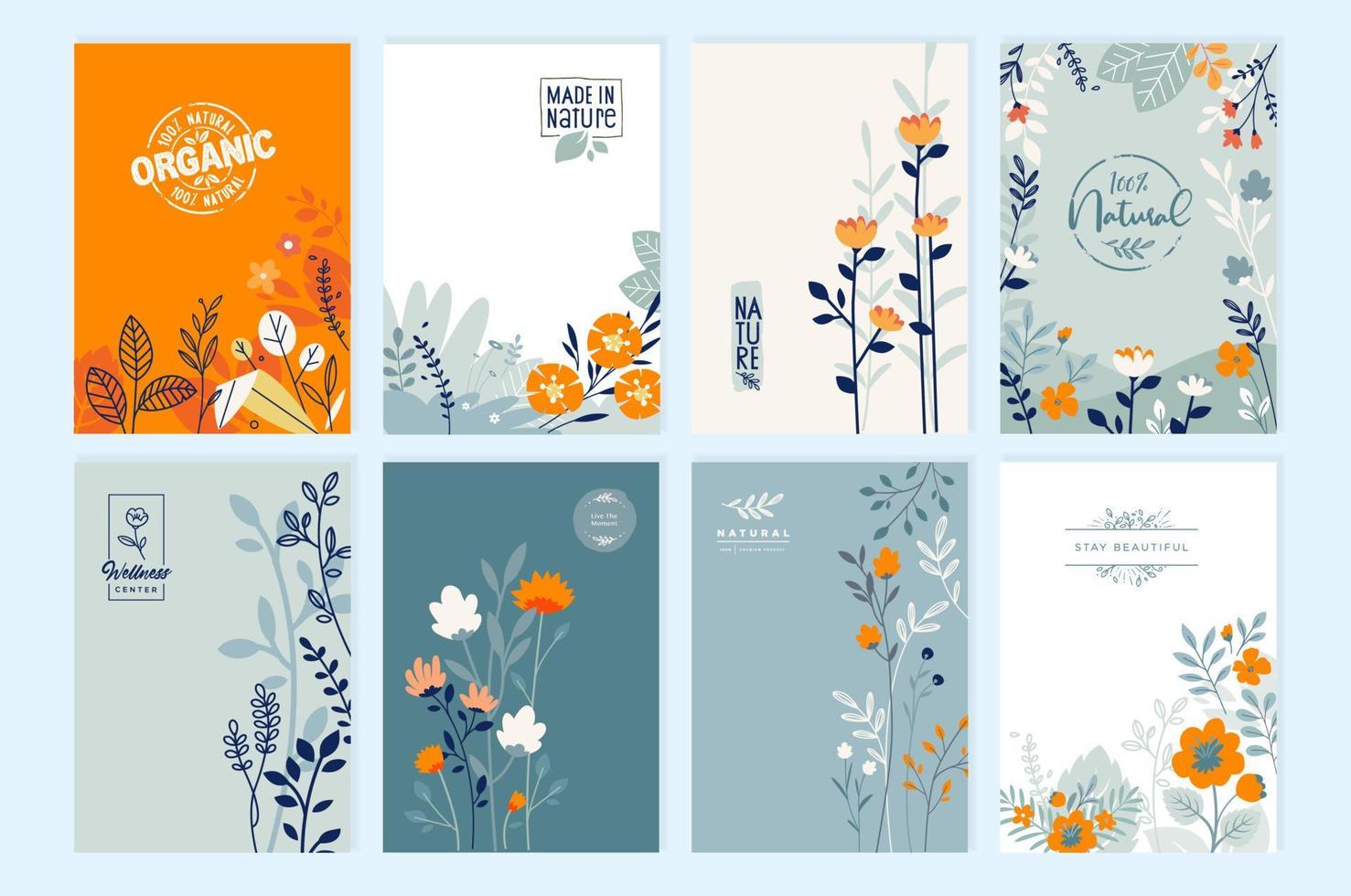This digitally synthesized image features eight rectangular greeting card designs arranged in two rows against a light blue background. The cards showcase colorful, clipart-style flowers in shades such as light gray, orange, blue, dark blue, light pink, and white, with varying backgrounds and orientations of floral designs.

In the top row, the first card, with an orange background, displays a circular graphic that reads "100% Natural" and "Organic" in white text. The second card has a white background with small flowers at the bottom and the phrase "Made in Nature" in dark navy within a small rectangle at the top. The third card, set against a cream-colored background, features tall, orange flowers with dark turquoise stems on the right side and the word "Nature" in dark blue, split into three lines: "NA," "TU," and "RE." The fourth card has a light sage green background with a floral border, and "100% Natural" written in darker green in the center.

In the bottom row, the first card shares the same dark green background as the fourth card above, presenting blue flowers on the right side and the text "Wellness Center" in navy script within a rectangle on the left. The second card has a dark teal background with peach-colored, white, and green flowers at the bottom left, displaying the small text "Live the Moment" in the top right corner. The third card, with a light gray background, features flowers in the same colors as the others and the word "Natural" in white text at the top left. The fourth and final card in the bottom row has a white background with flowers in gray, orange, and blue tones along the bottom, topped with the phrase "Stay Beautiful" in light gray.

Each card's distinct design, color scheme, and text contribute to an overall cohesive floral-themed collection, ideal for greeting cards or labels.